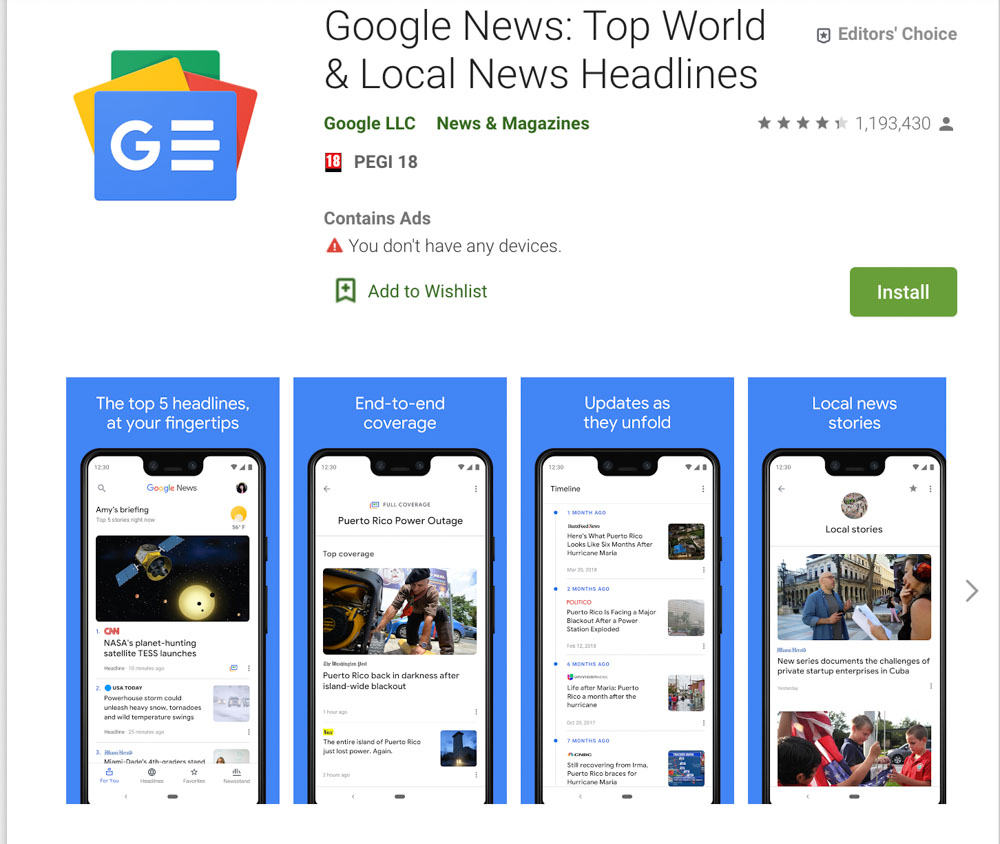The image displays a detailed page from the Google Play Store featuring an application for Google. The page resembles an advertisement, highlighting various functionalities and features of the app. Prominent icons in varying colors, some in green, add a visually appealing element to the design. Notable text includes an "Install" button accompanied by a note stating the app contains ads.

Beneath this section, the page showcases four phones, each displaying different aspects of the app interface, providing a visual preview of the user experience post-download. At the top of the page, bold text reads "Google News: Top World and Local News Headlines," indicating the app's primary focus. Additionally, the upper right corner features a label that reads "Editor's Choice," suggesting high editorial endorsement. The page also informs users that the app has been downloaded approximately 1,193,430 times, illustrated by a small icon of a person next to the download count.